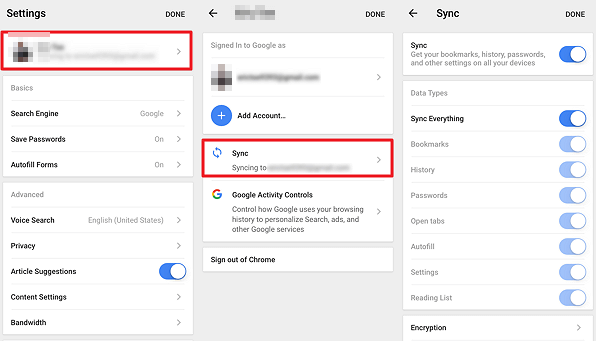This image is a composite screenshot, comprising three columns positioned adjacent to each other. Each column showcases different sections of a settings interface, with specific highlights and erasures made by the creator to draw attention to certain areas.

**First Column:**
- **Header:**
  - **Top Left:** "Settings"
  - **Top Right:** "Done"
- **Content:**
  - The section beneath this header is mostly erased but highlighted with a red border, indicating potential importance, though its exact detail is obscured.
  - **Highlighted Settings:**
    - **Basics:**
      - Search Engine: Google
      - Save Passwords: On
      - Auto-fill Forms: On
    - **Advanced:**
      - Voice Search: English
      - Privacy: Article Suggestions: On
      - Content Settings
      - Bandwidth

**Second Column:**
- **Header:**
  - **Top:** Back Arrow
  - **Right:** "Done"
- **Content:**
  - "Signed in to Google as" (with user information erased)
  - **Blue Button:** "Add Account"
  - A red mark emphasizes the section titled "Sync," but details about what is syncing are erased.
  - **Text:** "Google Activity Controls - Control how Google uses your browsing history to personalize search ads and other Google services."
  - **Option:** "Sign out of Chrome"

**Third Column:**
- **Header:**
  - **Top:** Back Arrow | "Sync"
- **Content:**
  - **Sync Description:**
    - "Get your bookmarks, history, passwords, and other settings on all your devices." (Sync is toggled On)
  - **Data Types:**
    - "Sync everything" (toggled On)

In summary, the image is a detailed view of a settings interface, with particular focus on key sections like "Basics," "Advanced," and "Sync." Specific settings such as default search engine, password saving, form auto-fill, and sync options are shown, though some user-specific information has been intentionally erased. The creator has highlighted areas of interest, especially in context with the synchronization and privacy settings.